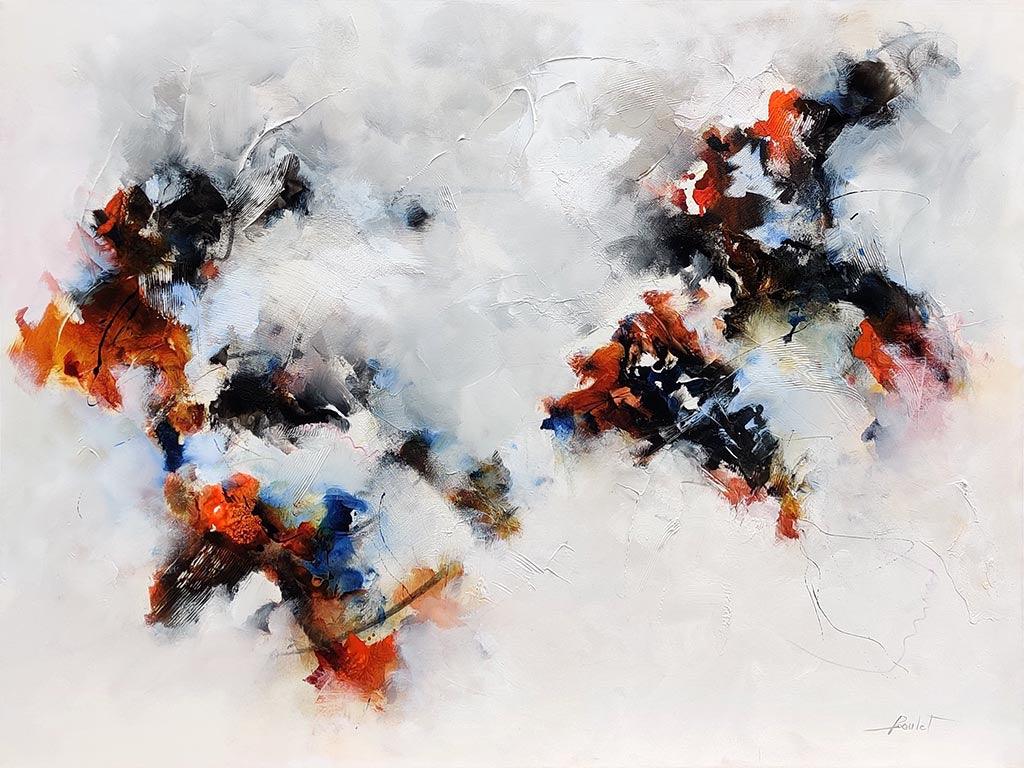This abstract painting features a captivating interplay of textures and colors. The background is primarily a light gray with hints of darker gray splotches, complemented by subtle white and beige areas that create a modern yet timeless ambiance. At the center of the artwork, two distinct shapes stand out, adorned with vibrant hues of orange, red, blue, white, and specks of black and gold.

The shape on the left resembles a stylized "E" with what appear to be three legs and a long nose-like extension. On the right, the shape recalls an "M" with leg-like protrusions at the bottom and a smaller head at the top. The colorful areas are strategically placed on the left and right sides of the canvas, leaving the middle relatively blank except for a single black dot that draws the eye. The dynamic paint strokes add depth and movement, showcasing shades of light blue, burnt orange, and black. This abstract piece blends the essence of modern art with a sense of aged sophistication, offering a rich visual experience.